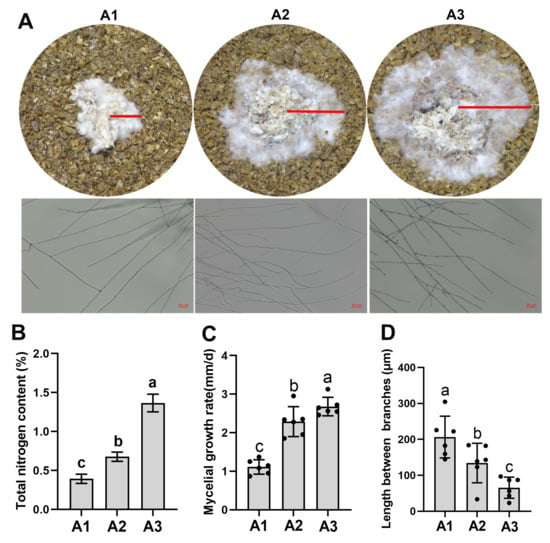The scientific diagram illustrates the progression of mycelial growth over three stages labeled A1, A2, and A3. At the top, three circular photographs showcase the mycelial growth on a brown-gray vermiculite-like background, increasing in size from left to right. Each image displays fuzzy white and gray mold-like growth at the center, with a small red line marking the radius from the center to the edge. Below these photographs, three gray rectangular images depict microscopic views of thin black filaments corresponding to the surface growth in the photographs above. At the bottom, three bar graphs labeled B, C, and D measure key parameters for each stage: total nitrogen content (in percent) for A1, A2, and A3, mycelial growth rate (in millimeters per day), and the length between branches (in micrometers). The diagram provides a comprehensive view of the experiment's findings, documenting the morphological and quantitative changes in the mycelial growth across the three stages.